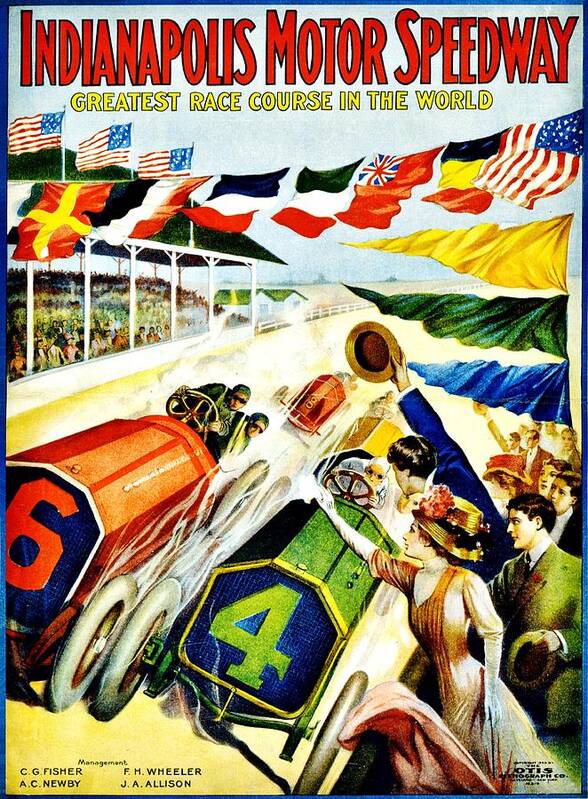This vibrant and nostalgic image depicts an old-era, colorful magazine cover or poster for the Indianapolis Motor Speedway. Dominated by a blue border, the top of the cover features bold red text with a black outline declaring “INDIANAPOLIS MOTOR SPEEDWAY” in uppercase letters. Below, smaller yellow text with a black outline proclaims it as the “GREATEST RACE COURSE IN THE WORLD,” also in uppercase. The imagery, which resembles a stylized painting, showcases the early 1900s racecars in action. Two prominent cars, a red one marked with a large orange number 6 and a green one with a green number 4, speed around the track, emitting billowing smoke from their tires. The scene is bustling with spectators—men and women donned in 1930s-style attire—crowded to the right side and on the bleachers to the left. American flags—red, white, and blue—along with numerous other international flags such as Germany, Italy, and Britain, flutter from strings above, adding to the sense of a grand, global event. The background features a green hill under a blue sky, enhancing the lively and competitive atmosphere of this historic race scene.